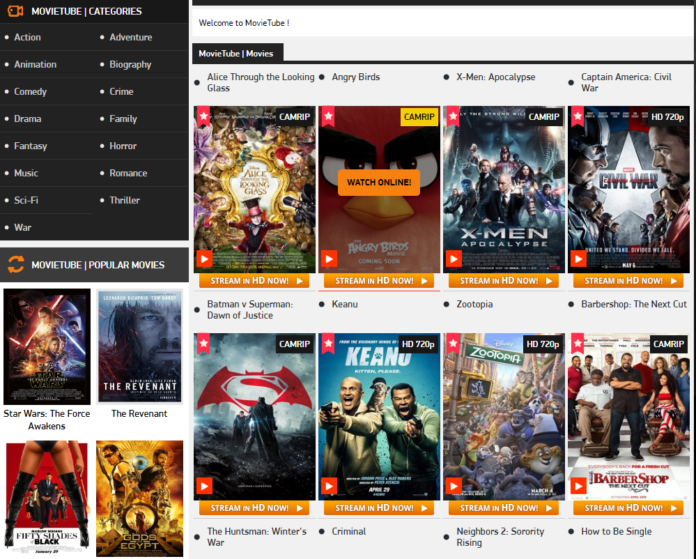The interface displays a vertical, black sidebar on the left side, topped with a red icon representing a video camera. Adjacent to this icon, a label reads "MovieTube," followed by a small vertical divider and the word "Categories."

The categories are organized into two vertical columns. The left column includes:
- Action
- Animation
- Comedy
- Drama
- Fantasy
- Music
- Sci-Fi
- War

The right column lists:
- Adventure
- Biography
- Crime
- Family
- Humor
- Romance
- Thriller

To the right of the categories, several movie options are displayed. The first row of movie choices includes:
1. **Alice Through the Looking Glass**: Featuring Johnny Depp as the Mad Hatter with red hair and a tall hat.
2. **Angry Birds**: Displayed in the background with a prominent "Watch Online" button in an orange box at the center.
3. **X-Men Apocalypse**.
4. **Civil War**.

The second row below showcases:
1. **Superman**: Identified by the iconic 'S' symbol within a diamond.
2. **Keanu**: Depicting two men holding guns, their mouths open in expression, one with a doll perched on his shoulder.
3. **Zootopia**: Filled with various animated characters.
4. **Barbershop**: Featuring a large group of people standing on a black and white checkered floor, accompanied by an orange box reading "Stream in HD now".